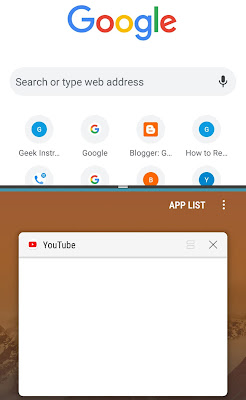The image appears to be a screenshot of a cell phone screen, which is much taller than it is wide. The screen is divided into two main sections: a top area with a white background and a bottom area.

At the very top, the word "Google" is displayed in a colorful font: the two G's are blue, the first O and the E are red, the second O is yellow, and the L is green. Beneath this, there is a gray search bar that reads "Search your type address" with a microphone icon on the far right.

Below the search bar, there is a row of icons. The first four icons read "Geek," "INSTR…" (partially obscured), "Google," and "Blogger." Following these, there are two more partially obscured icons: one reads "G…" and the other "How to, RE…"

Another row of icons is partially covered by another image overlay. The visible icons in this row include a phone icon, another Google icon, a circle with an orange background and a B in the middle, and a blue circle with a Y in the middle.

In the second half of the screen, towards the bottom, there is a section with an orange background that says "App list" in the top right corner. This area is mostly covered by a white square overlay. This overlay has a light gray top border, and in the top left corner, it says "YouTube."

Overall, the image is a detailed view of a smartphone interface, featuring a Google search bar, several app icons, and a partially covered section displaying the YouTube app.